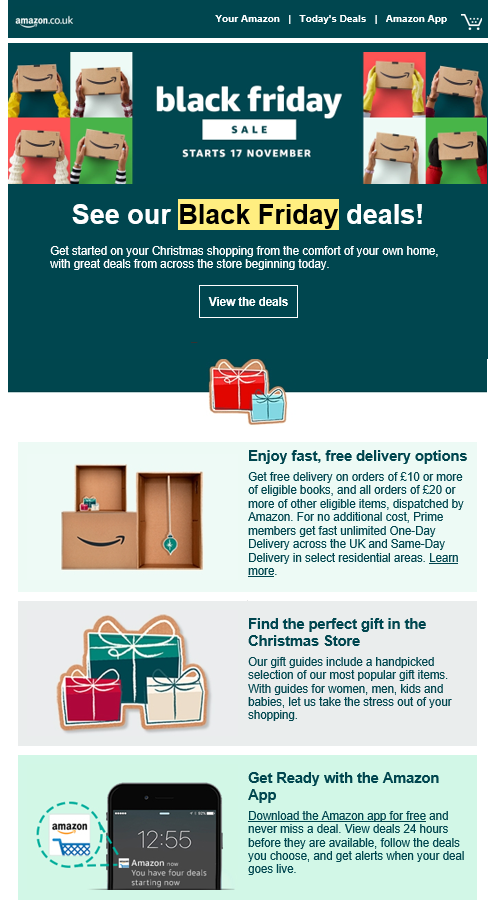The image is a screenshot from the Amazon UK website during a promotional period. At the very top of the page, there's a navigation bar showing "amazon.co.uk," with options such as "Your Amazon," "Today's Deals," the "Amazon App," and a small shopping cart icon.

The central section of the image prominently features multiple hands of varying sleeve lengths and backgrounds, each holding an Amazon box, symbolizing diversity and inclusivity. A banner text states, "Black Friday sale starts 17th of November. See our Black Friday deals," suggesting customers can start their Christmas shopping early with impressive discounts. A clickable button labeled "View the deals" is prominent for easy navigation.

Below this, there are two boxes wrapped as Christmas presents, accompanied by the text promoting free delivery options. It highlights that customers can enjoy free delivery on eligible book orders over £10 and other items over £20. Prime members are additionally entitled to fast, unlimited one-day delivery across the UK and same-day delivery in select residential areas. There is an image of an Amazon box with a hanging ornament nearby.

Further down, a section encourages users to "Find the perfect gift in Christmas Store," featuring guides for various demographics—women, men, kids, and babies—designed to simplify the shopping experience with a curated selection of popular gift items.

Lastly, the image advertises the Amazon App, encouraging users to download it for free to ensure they "never miss a deal." The app provides features like viewing deals 24 hours in advance, following selected deals, and receiving alerts when a deal goes live.